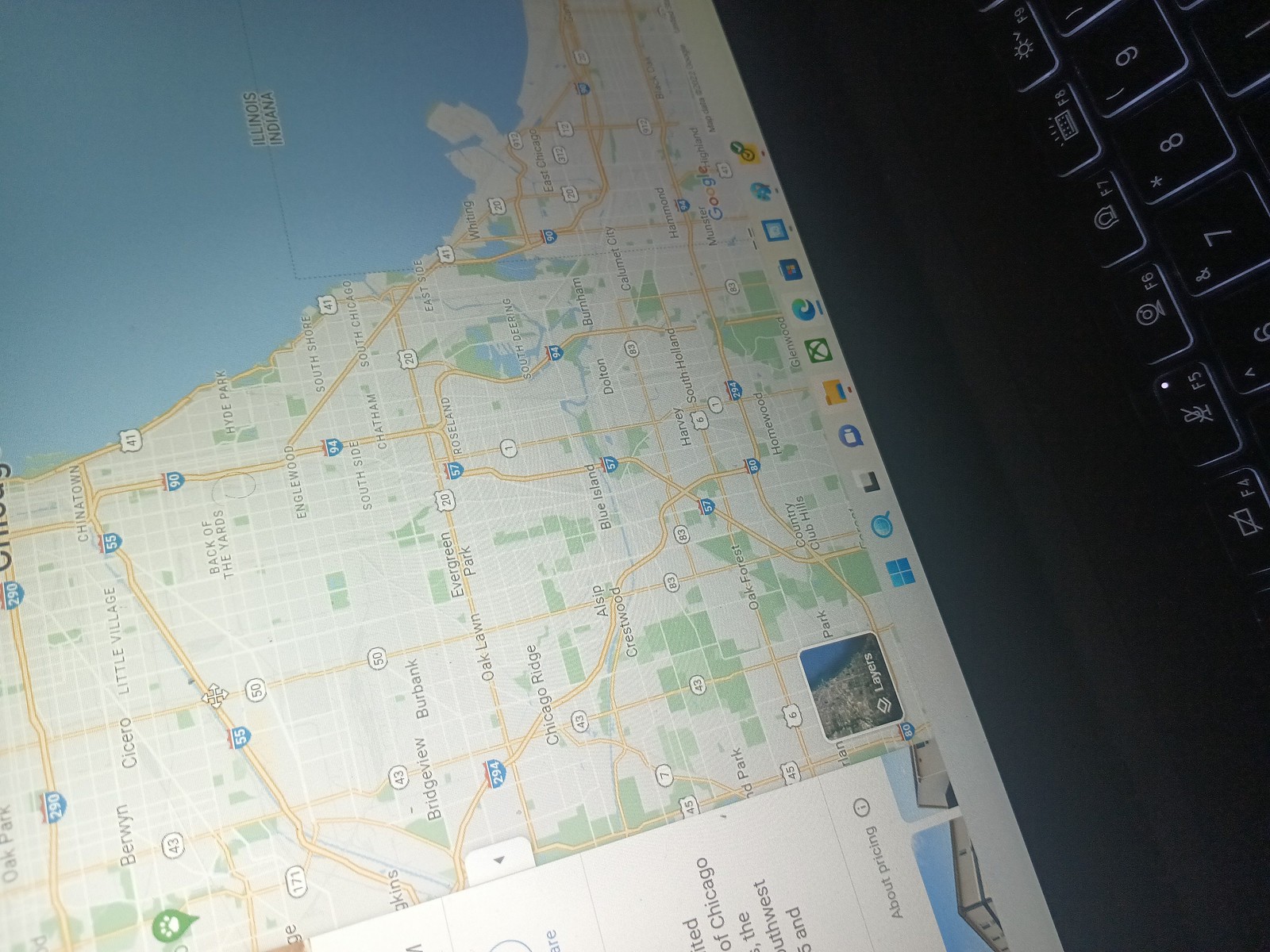This is a detailed close-up image of a laptop that's been turned sideways, providing a unique perspective. The laptop's screen displays Google Maps, showing various locations such as Evergreen Park, Burbank, Chicago Ridge, and Oak Lawn Park, with a visible body of water in the top left corner. The laptop itself has a black keyboard, and you can see the top row of number and function keys prominently in the upper right corner of the image. The taskbar at the bottom of the screen features a Windows icon, an Xbox icon, and several other icons, indicating it is a Windows computer. Although the image was likely taken accidentally, it provides a clear and detailed sideways view of both the map on the screen and the top part of the keyboard.